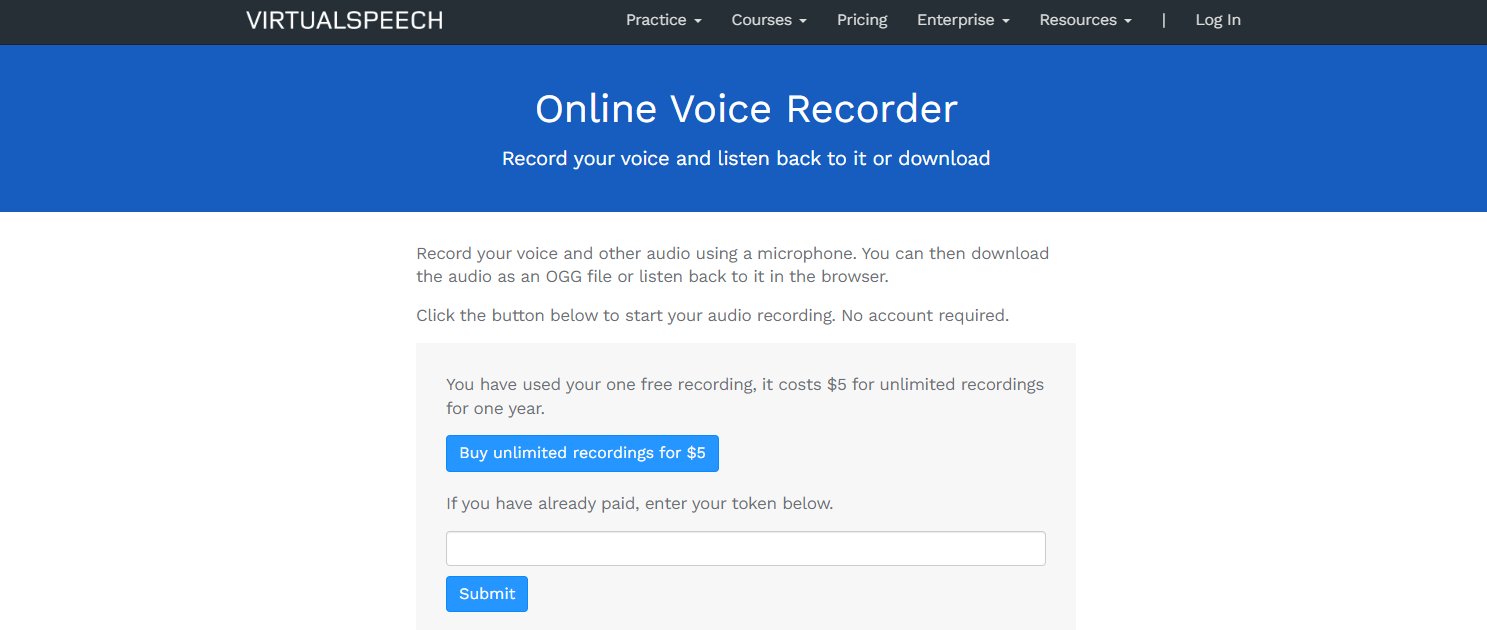Here is a detailed and cleaned-up caption for the image described:

---

The screenshot displays a website featuring a structured interface aimed at voice recording services. At the very top, there's a black navigation bar with white text, listing options from left to right: "VirtualSpeech," "Practice," "Courses," "Pricing," "Enterprise," "Resources," and "Login." 

Below the navigation bar, a prominent purple rectangle with white text announces "Online Voice Recorder - Record your voice and listen back to it or download".

Directly below this, the main content area of the page features a clear white background with informative text in black font: "Record your voice and other audio using a microphone. You can then download the audio as an OGG file or listen back to it in the browser. Click the button below to start your audio recording. No account required."

Further down, a gray rectangle with black text informs users: "You have used your one free recording. It costs $5 for unlimited recordings for a year."

Beneath this message, a blue button with white text accommodates users wishing to purchase unlimited recordings: "Buy unlimited recordings for $5."

Additionally, there is a prompt for those who have already made a purchase: "If you have already paid, enter your token below." This instruction is followed by an empty white text field for token entry, and a supportive blue button with white text labeled "Submit."

---